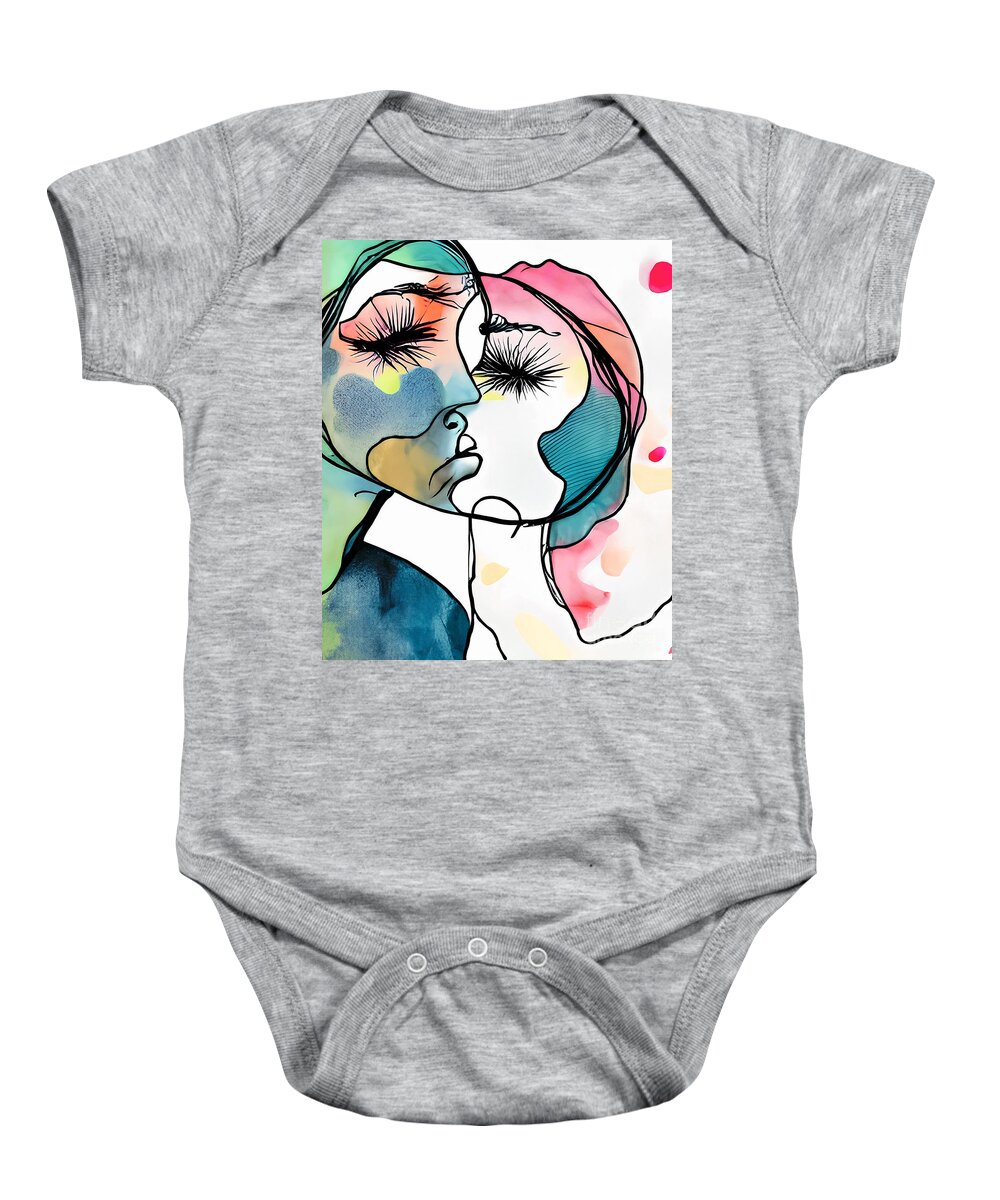Displayed against a white background, this baby onesie is crafted from soft, heathered gray cotton, ensuring comfort for the little one. The onesie features three buttons at the bottom, making it easy to slide over the baby's head and secure over a diaper. Prominently displayed in the center is an abstract, iron-on artwork depicting two people, appearing to be women, in a tender kiss. Their faces merge into one another in a modern, watercolor style, blending a palette of bluish greens, yellows, reds, pinks, and oranges. The intertwined faces are adorned with fluffy black eyelashes and are detailed with a multi-lined starburst effect where their eyes should be, creating a striking and artistic centerpiece on the garment.